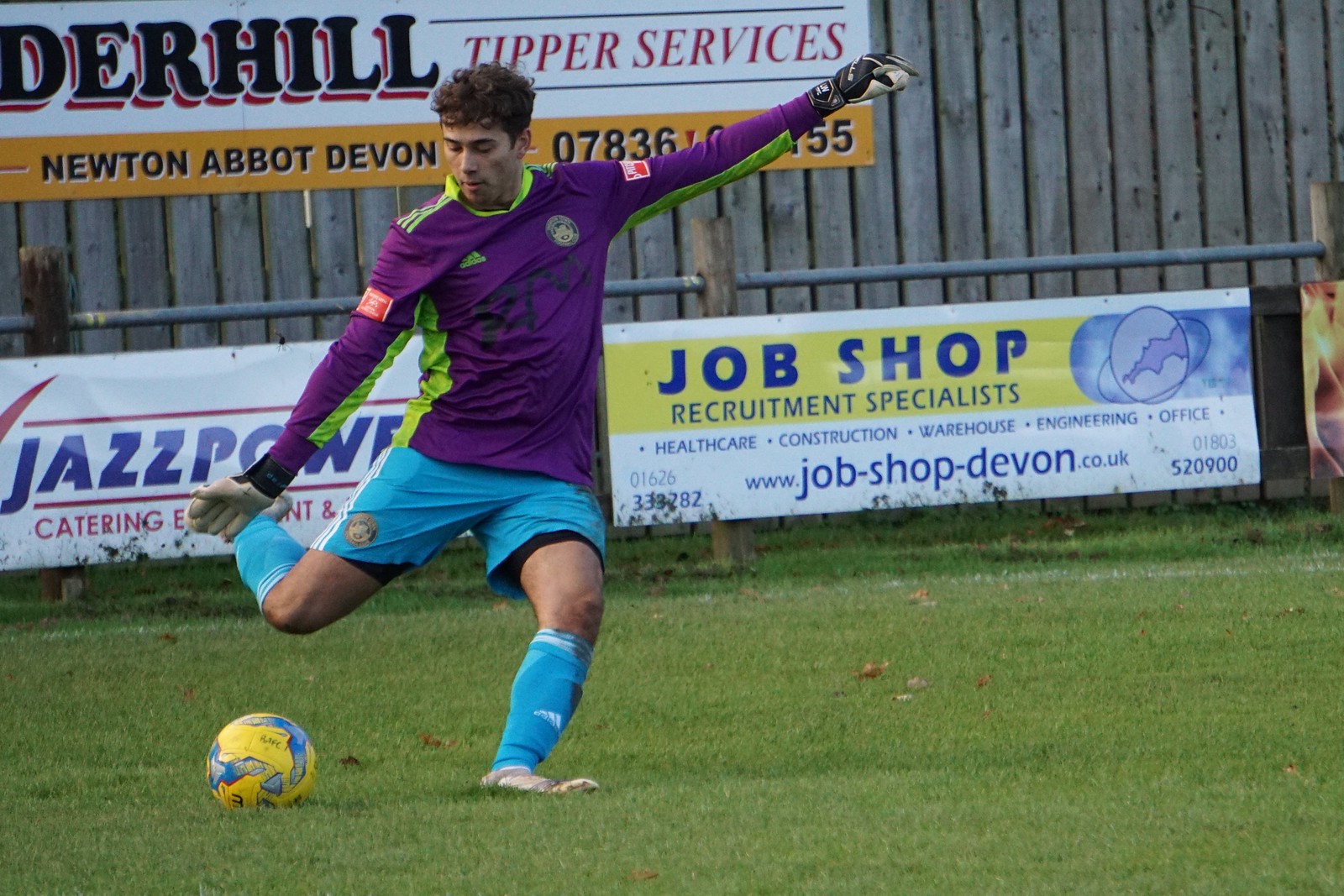In this landscape-oriented photo of a soccer game, the backdrop features a gray wooden fence adorned with various promotional signs. One prominent sign reads, "Something Hill Tipper Services and Whites," with a yellow stripe below bearing the text "Newton Abbott Devon" and an unreadable phone number. In front of this wooden fence, there's a smaller wooden-metal fence displaying more vinyl signs. One advertises "Jazz Power and Whites" catering services, and another promotes "Job Shop Recruitment Specialists."

The foreground is dominated by a well-trimmed grass soccer field. A white player with slightly curly, short hair is prominently positioned, poised to kick a yellow soccer ball. Dressed in a purple jersey, bright blue shorts, and matching blue socks, he also wears gloves, suggesting he is the goalkeeper. His focused stance indicates he is about to deliver a powerful kick.